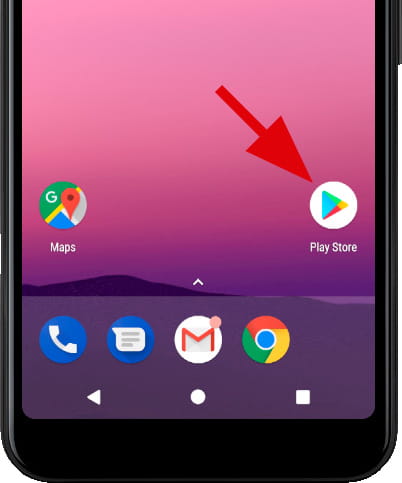This screenshot captures the lower half of a smartphone display featuring a vivid and colorful background that transitions from pink to purple, with a stylized mountain range at the bottom. Dominating the image is a large red arrow pointing to the Play Store icon, which is centrally placed on the right side of the screen. The Play Store icon itself is a white circle containing a multicolored triangle—blue, red, green, and yellow—pointing to the right, with the label "Play Store" beneath it.

On the left side of the screen, the Google Maps icon is prominently displayed, showcasing a graphical rendition of a map in Google's signature colors: a red pin, a blue shape, a yellow marking, and a green area representing land. This icon features a white "G" within the red pin, which resembles an upside-down teardrop with a black circle in the center.

Towards the bottom of the image, near the mountain range, there is an upward-facing arrow suggesting that an additional menu can be accessed by swiping up. A semi-transparent rounded rectangle, located in the bottom center of the screen, houses four distinct icons: a white telephone on a blue background, an upside-down speech bubble with gray rectangles inside a blue circle, a white circle with a red-outlined envelope that forms the letter "M" indicating new mail, and the familiar multicolored Google icon, which is a smaller blue circle encircled by white, and surrounded by yellow, red, and green segments.

Lastly, the very bottom part of the phone screen displays the navigation bar, featuring three standard Android navigation icons: a triangle pointing left (Back), a circle (Home), and a square (Recent Apps).